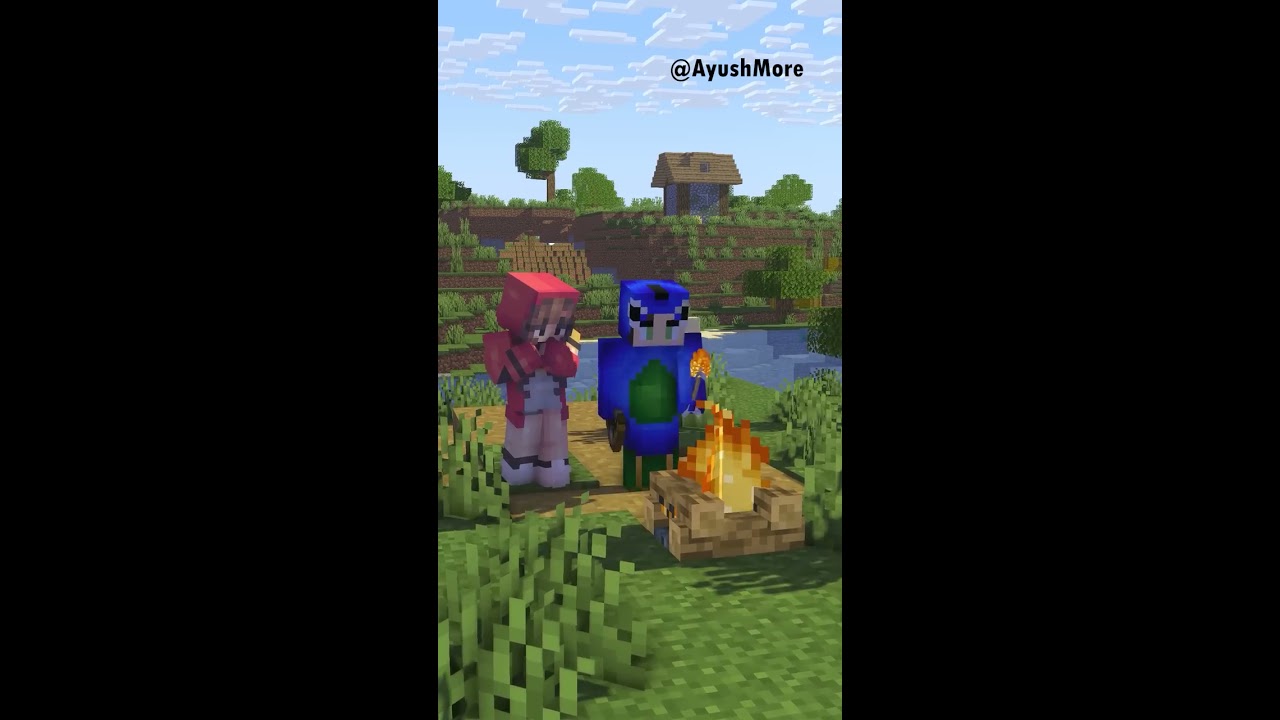In this color screenshot taken from a 3D game that bears a striking resemblance to Roblox or Minecraft, the scene is vividly detailed. The background features a blue sky dotted with white clouds, terraced land, and a blue cottage with a brown roof nestled among the trees. The terrain consists of blocky, pixelated dirt and grass, with a body of water in the midground contributing to the tranquil setting. In the foreground, two robot-like characters are attending to a campfire, which burns red and yellow in a brown fire pit. One character is dressed in a red hoodie and small shoes, while the other sports a combination of blue, black, and white with a distinctive green chest. They appear to be cooking marshmallows. The entire scene is wrapped in white and black bands on the sides of the image and features a watermark in the upper right corner with the text "@Ayushmore."